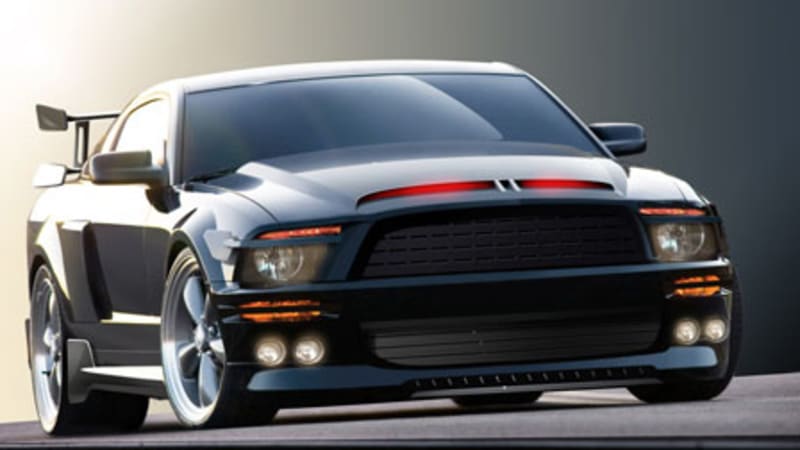This image depicts a high-end sports car, possibly a Ford Mustang, on a gray asphalt surface. The car appears impeccably new and exhibits a dynamic, rugged design. It features a black or navy blue exterior that is highly reflective, giving it a shiny appearance. The car's front is adorned with red stripes near the grille and flanked by distinctive white and orange lights, while the rear of the vehicle showcases a dark gray color. Notably, the car includes a rear spoiler and sports silver wheels, indicating its high-performance nature. The background is a gradient that transitions from white on the left to gray on the right, suggesting an abstract or digitally altered setting. The scene is devoid of people, emphasizing the car's sleek and powerful design, and the light source appears to be coming from the left, casting bright highlights and creating a dramatic effect.